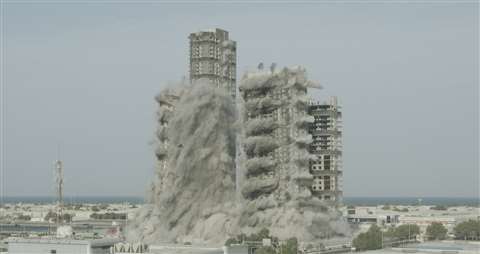The image captures a dramatic scene of two tall buildings being imploded. The building on the left, which is cylindrical and lined with windows, is already cascading downward, enveloped in large plumes of gray concrete smoke billowing out from the bottom and sides. The structure on the right, shorter and with visible railings on its sides, is also in the process of collapsing, with smoke rising from each level as it comes down on itself. In the distance, a range of hills transitions into a cityscape of small white buildings, adding depth to the mid grayish-blue overcast sky. The background also features a beach and ocean, providing a stark contrast to the chaos of the implosion. Decorative trees line a concrete area on the left corner of the image, while a line of bushes is visible on the right side near the corner, framing the scene and adding elements of tranquility amidst the destruction.